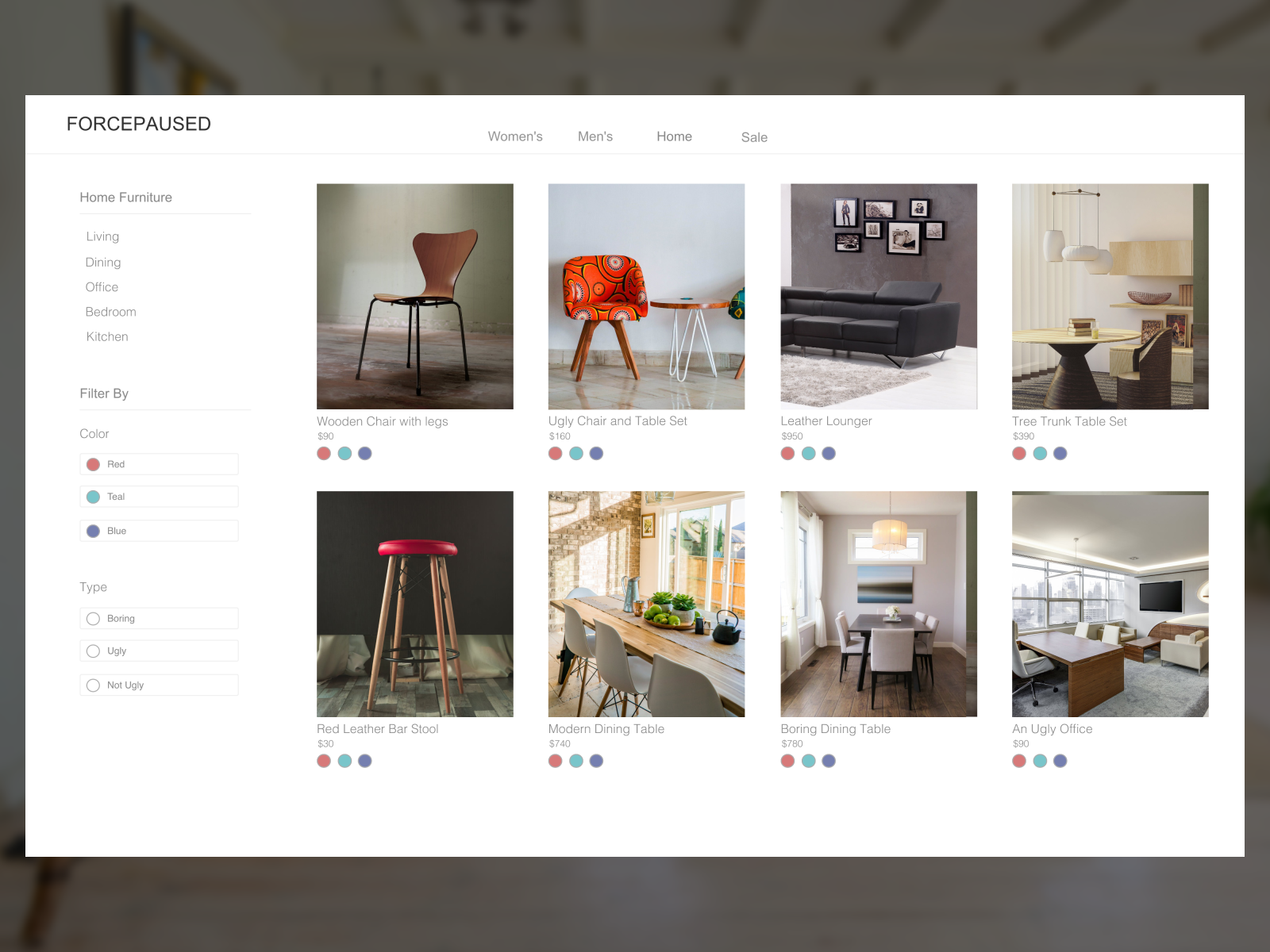In this image, we see a section of an online furniture store's interface, showcasing a variety of home furnishings. The page is divided into tabs for different categories such as "Women's," "Men's," "Home," and "Cell." Along the left side, there are filter options for different furniture categories like "Living," "Dining," "Office," "Bedroom," and "Kitchen," as well as filters by color (red, teal, blue) and type (boring, ugly, not ugly), although none of the checkboxes are selected.

The main content area is organized into a 4x2 grid displaying various furniture items:

1. A wooden chair with legs available in red, green, and blue, priced at $90.
2. An unattractive chair and table set priced at $160, available in red, teal, and blue. The chair is orange, and the table is small.
3. A leather lounger priced at $950, available in red, teal, and blue.
4. Paintings on the wall and a tree trunk table set, which includes a table and chair designed in a tree trunk style.
5. A red leather barstool, showcased against a black wall.
6. A modern dining table priced at $740, which includes a wooden table and some chairs with glass walls in the background.
7. Another modern dining table setting, featuring a wooden table and chairs.
8. An unattractive office setup priced at $90.

Each item is vividly detailed with color options and pricing, giving potential buyers a clear view of the available selections.